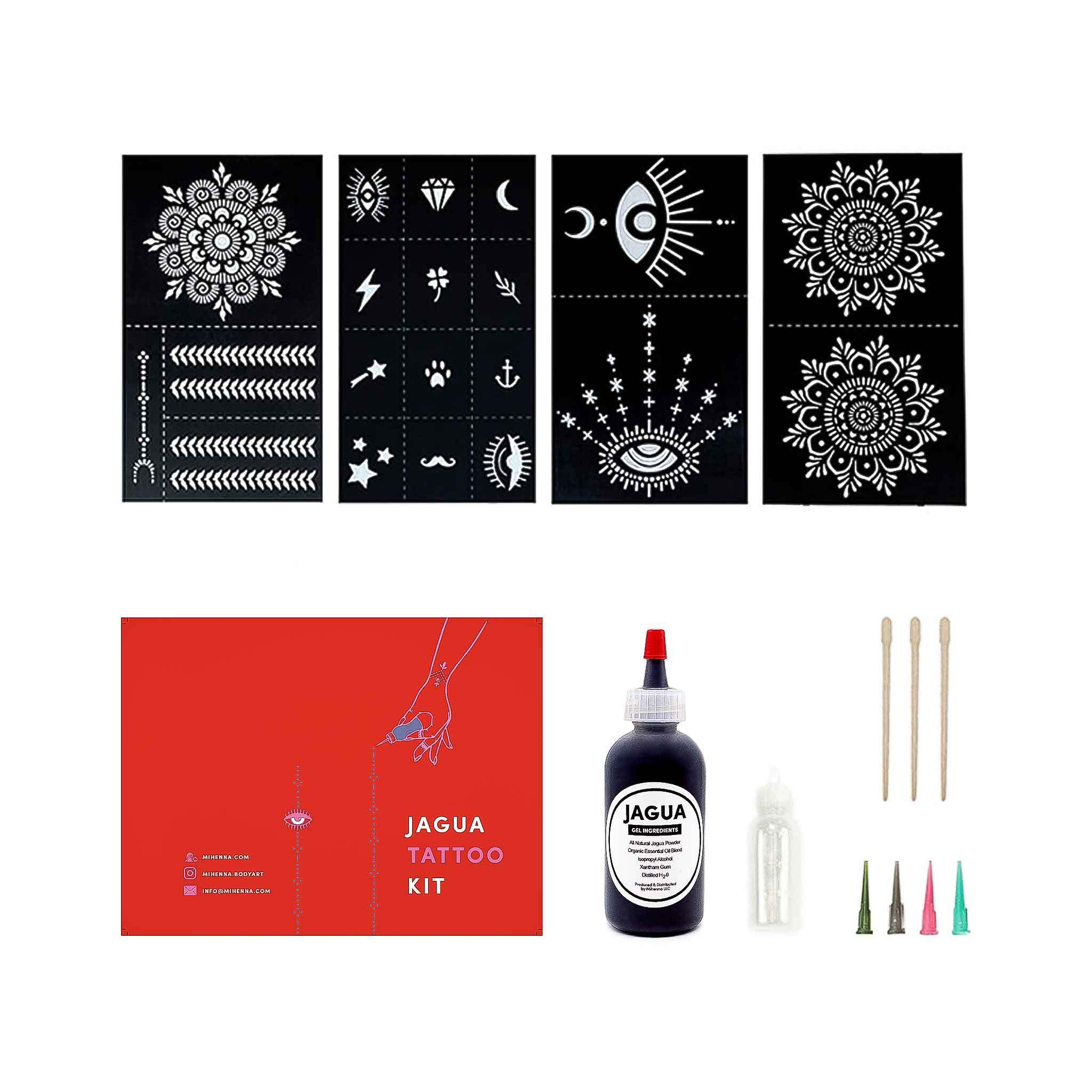The image showcases a detailed advertisement for the Jaguar Tattoo Kit, which appears to be a temporary tattoo set resembling henna. The lower left corner features a prominent red rectangle with a blue illustration depicting a hand squeezing a bottle of ink along a line, while another line with an eyeball design is visible to its left, both accompanied by unreadable small text. Central to the image is a large black ink bottle labeled "Jaguar" in bold black text, topped with a red cap, akin to a condiment bottle. Adjacent to it is a smaller unlabeled white or gray bottle blending into the background, and next to these are three wooden dowels. To the right of the dowels, there are four interchangeable colored tips—green, greenish-gray, pink, and blue-green—presumably for varied ink flow regulation.

Dominating the top part of the image are four stencil sheets in black and white, featuring an assortment of intricate and decorative tattoo designs. These include mandalas, floral patterns, various small symbols like an eyeball, a diamond, a crescent moon, a lightning bolt, a four-leaf clover, a grain of wheat, a magic wand, a paw print, an anchor, stars, a mustache, and some uniquely elaborate eyeball designs. The designs seem to serve as guides for applying the tattoo ink to the skin, offering an array of creative temporary tattoo possibilities. Each sheet is densely populated with these detailed, India henna-style patterns, set against a black background and separated into four sections, possibly indicating multiple stencils per sheet for versatile use.